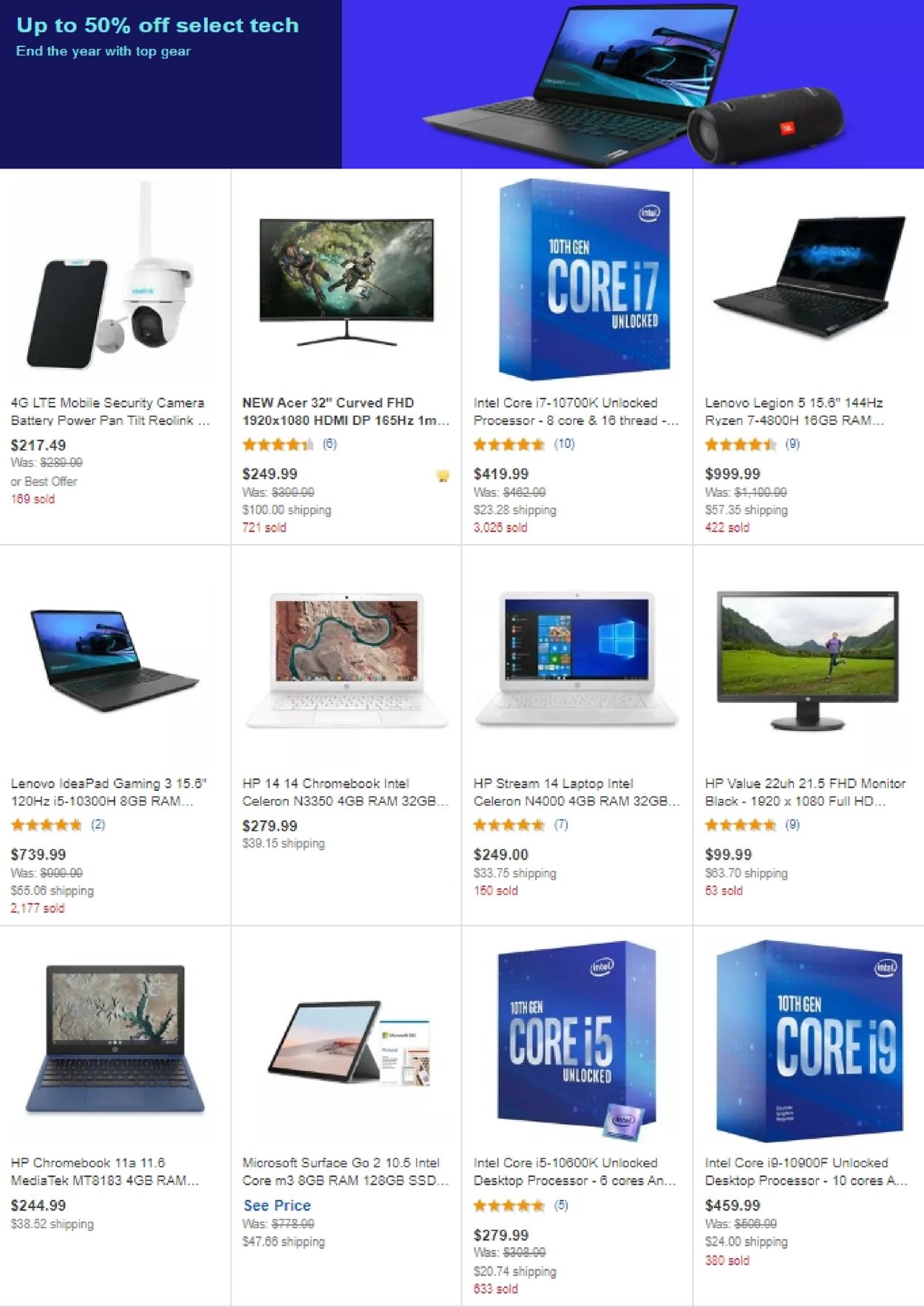The webpage displays a selection of electronics without a clear store title. At the top left, a small placard announces "Up to 50% off select tech." On the right, there's an image featuring an open laptop and a professional camera lens. Below the top banner, twelve items are arranged from left to right, each accompanied by a description and price. 

On the left, the first item is a 4 LTE mobile security camera from Ring, priced at $217.49. Next is an Acer 32-inch curved television screen, available for $249.99. Further down, an HP Chromebook is displayed with a price tag of $244.99. 

The very last item, located in the bottom right corner, is an Intel Core i9 10th generation desktop processor, showcased in blue and priced at $459.99. Each product listing is detailed, offering potential customers a clear view of the offerings.